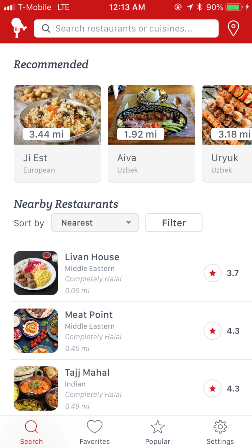The screen displays a T-Mobile LTE signal with a 90% battery life, captured at 12:13 a.m. It suggests recommended GE East directions with a distance of 3.44 miles, and other locations AVA at 1.92 miles and Eurek at 3.18 miles. 

Nearby restaurants are sorted by proximity, including:
- "Live in House," a Middle Eastern restaurant with a 3.7-star rating.
- "Meat Point," another Middle Eastern restaurant rated 4.3 stars.
- "Taj Mahal," an Indian restaurant also rated 4.3 stars.

The interface includes options to search favorites and access popular settings. Displayed at the bottom are three images of food plates adorned with items in various colors including orange, red, green, yellow, and brown. At the top, another set of three plates can be seen with similar items, except the rightmost plate features neatly lined-up bread rolls.